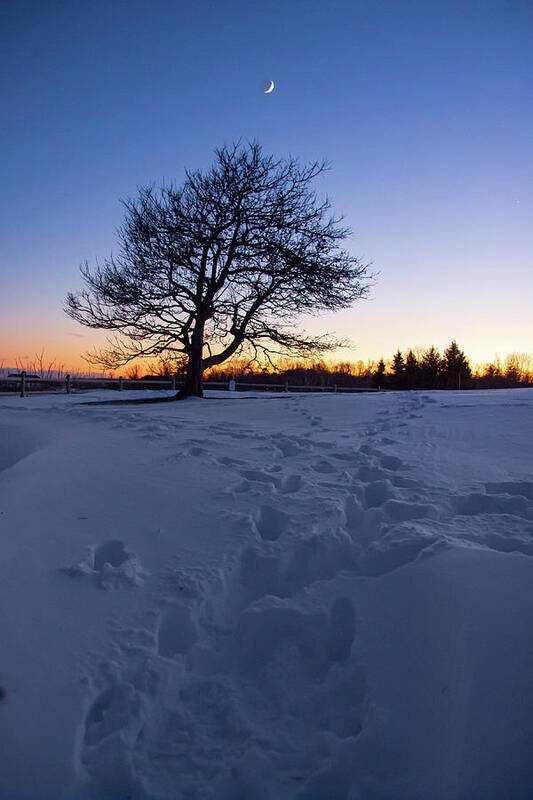This captivating image depicts a serene snow-covered field at dusk with a well-trodden trail created by at least two people walking side by side. Dominating the left side of the picture is a lone, leafless tree standing prominently against the wintry landscape. In the distance, the evergreen trees are bathed in the soft glow of a setting sun, casting a warm and beautiful light across the scene. A wooden fence extends from the left to right toward the background, enhancing the rustic charm of the scenery. Above, the sky retains a hint of blue, with a crescent moon beginning to shine, adding a tranquil touch to the snowy field. The snow itself appears to be quite deep, undisturbed except for the footprints leading towards the solitary tree, suggesting a peaceful evening slowly transitioning into night.